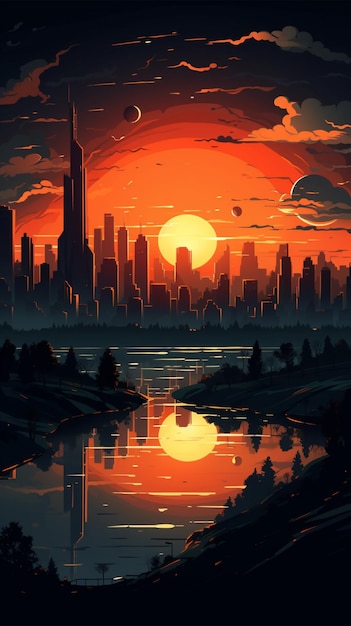The illustration depicts a stunning, computer-generated futuristic city skyline at sunset. Dominating the horizon is a prominent skyscraper with a pointed top, rising above a cluster of other gleaming buildings. The setting sun casts an orange-red glow across the entire scene, creating a moody and atmospheric ambiance. The sky is filled with clouds that take on progressively darker shades of orange and red as they stretch outward from the bright yellow sun. Adding to the sci-fi feel are additional celestial bodies, including a sliver of a crescent moon and possible planets that enhance the surreal quality of the sky. 

In the foreground, a body of water spans roughly fifty percent of the image, mirroring the striking skyline and the vivid colors of the sunset, as well as the celestial phenomena and clouds above. Tree-lined banks frame this body of water, contributing a natural element to the otherwise urban scene. The water appears to be composed of two distinct sections connected by a narrow channel, adding depth and complexity to the overall landscape. The entire color palette oscillates between dark blacks and grays, contrasted sharply by vibrant yellows and oranges, making for a visually captivating and immersive image.